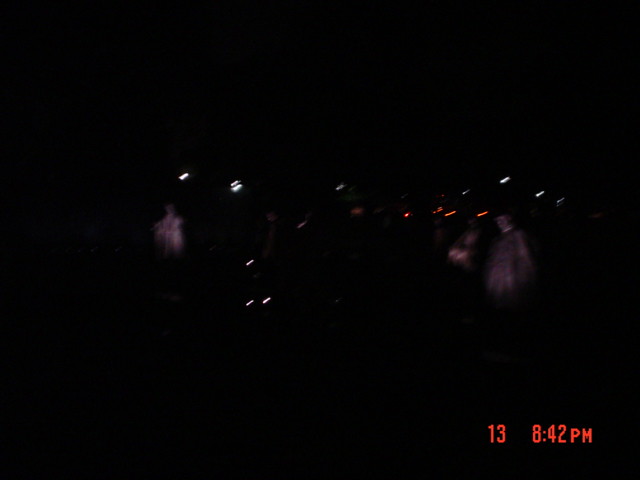The photograph is a dimly lit scene, seemingly from a Halloween exhibition. The backdrop is pitch black, enhancing the eerie ambiance of the setting. Positioned in the frame are four spectral figures, seemingly ghoulish apparitions donned in long, vintage attire reminiscent of the 1800s. Two of these figures are on the left side of the photo, and two are on the right, each exuding a haunting presence. A curious mix of red and white light flickers in the middle of the image, adding to the ghostly atmosphere. The photograph appears to be taken at night, as indicated by the vivid red timestamp at the bottom right corner, displaying "13" and "8:42 PM" in bright red digits.